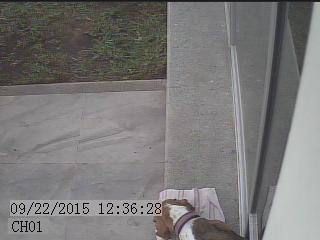The digital surveillance footage, captured on 09/22/2015 at 12:36:28, shows a small dog with light brown and white fur situated in the bottom left corner of the wide rectangular image. The dog, wearing a multicolored collar, is lying on a white towel with purple stripes. To the right of the dog, the side of a house is visible, featuring a window. A gray paved ledge runs vertically along the image’s right edge, transitioning into a gray sidewalk made of square tiles starting just above the middle on the left side. Above the sidewalk, there is a patch of dirt interspersed with dark green grass. In the bottom right corner of the image lies a white package on the cement ground. The digital timestamp reading "09/22/2015 12:36:28" is displayed over a gray bar.